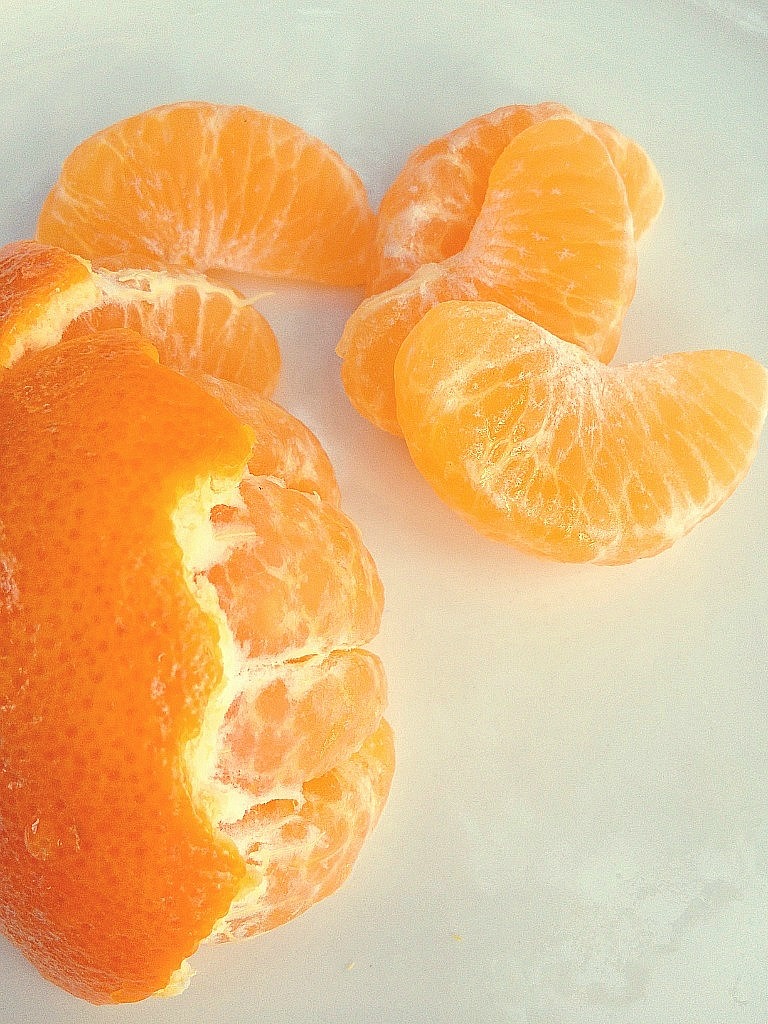The photograph features a close-up view of a small orange, partially peeled, situated on a plain white surface, likely a tabletop. The lower right corner of the image showcases half of the orange that still has its thick, vibrant orange peel attached, exposing the lighter-colored inner fruit. Four to five individual orange segments, varying in shades from light orange-yellow to darker orange and adorned with white lines, are scattered towards the top of the image. Among the peeled segments, one can spot a droplet of juice on the orange’s surface in the bottom left corner. The arrangement of the segments appears casually piled and positioned around the remaining half of the orange. Overall, the scene captures the fresh, juicy appeal of the orange against a plain white background, with no other objects visible.